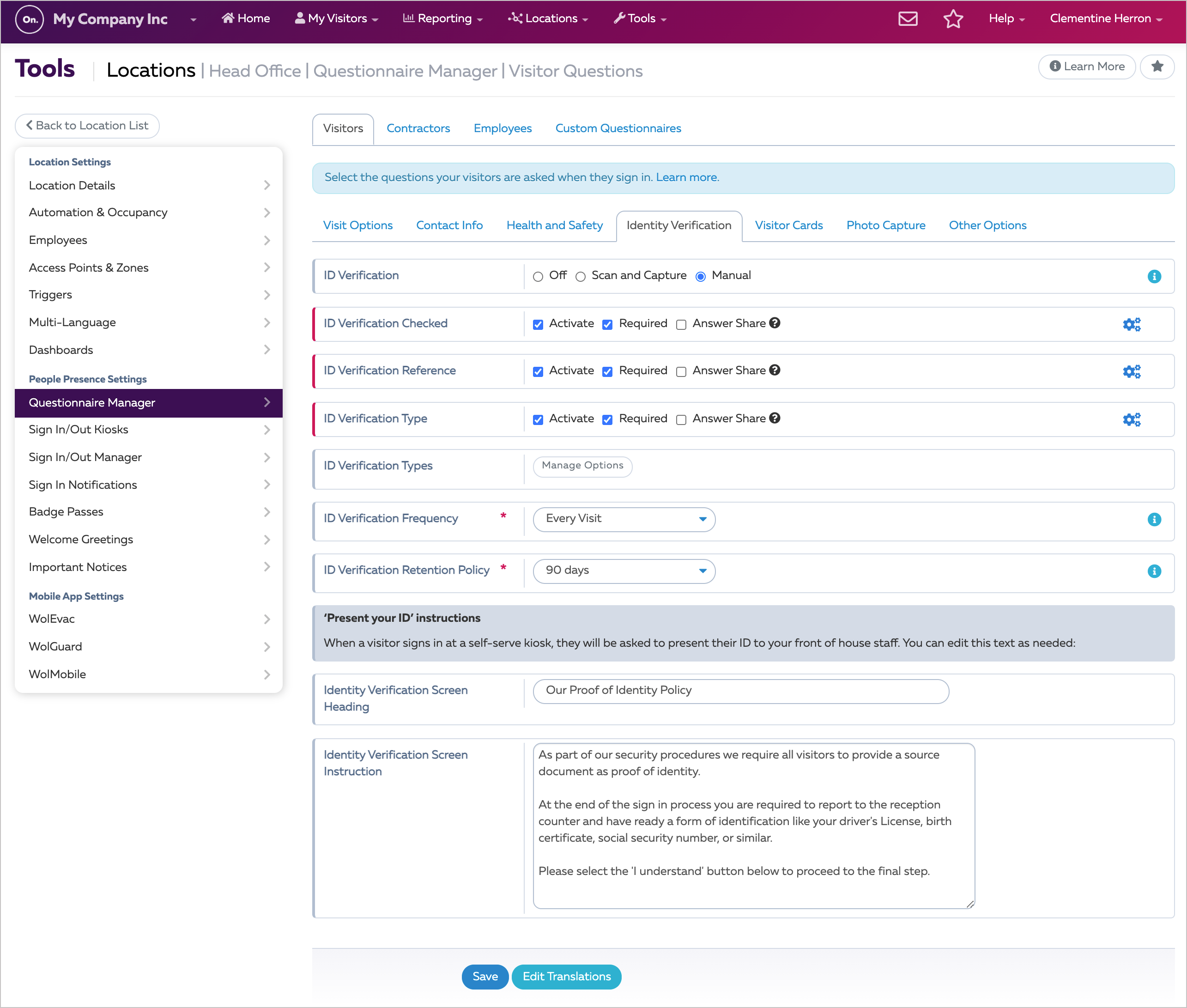**Detailed Description of Website Screenshot**

The screenshot showcases a section of a website with a clean, white background. At the very top, a dark blue navigation bar spans the width of the page. Displayed prominently in white font on this bar is the company name, "My Company INC." To the right of the company name are various navigation options starting with "Home," followed by "My Visitors," "Reporting," a "Locations" drop-down menu, a "Tools" drop-down menu, and a "Help" drop-down menu. The icons next to these options include an email icon and a five-pointed star icon. Furthest to the right, the current user is identified as "Clementine Heron."

Directly below the navigation bar, the main content area of the webpage begins. The heading "Tools" is displayed, alongside "Locations" and "Head Office." Beneath this, the page is further organized into sections such as "Questionnaire Manager" and "Visitor Questions." There are two buttons available for user interaction: one labeled "Learn More" and another featuring a five-pointed star icon.

On the left side of the webpage, a sidebar provides additional navigation options under the heading "Back to Location List." Below this, various clickable sections are available under the headings: 
- "Location Settings" 
- "Location Details"
- "Automation and Occupancy"
- "Employees"
- "Access Points and Zones"
- "Triggers"
- "Multi-Language"
- "Dashboards"
- "People"

The current selection in this sidebar is "Questionnaire Manager," which is highlighted with a black outline. Further down the sidebar, the labels "Present Settings" and "Sign In and Out Kiosks" are also visible, though they are not currently selected.